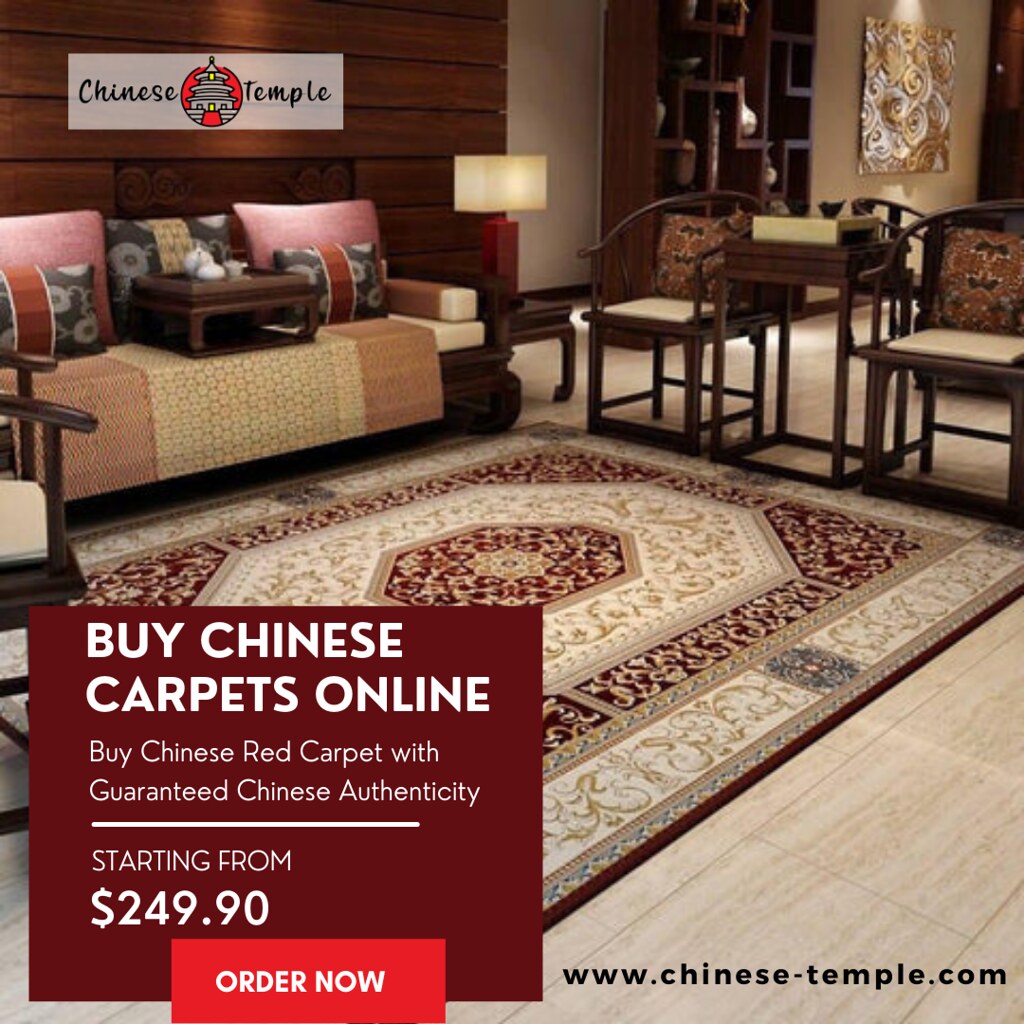This detailed catalog page appears to be from a carpet or furniture store, possibly the cover or an interior page. The main image showcases a showroom setting with a large, ornate Chinese carpet placed prominently in front of a couch and several chairs. There is a light-colored end table adorned with a lamp also in the scene. The carpet is richly decorated in red, beige, and gold, featuring intricate floral patterns. The room itself has a hard tile floor and a wooden texture on the walls, with some additional storage components and artwork visible in the background.

In the upper left corner of the page is the company's logo: a cartoon-like graphic of a Chinese temple positioned between the words "Chinese" and "Temple." Below, in the lower left, there's a brownish maroon background with white text that reads, "Buy Chinese Carpets Online. Buy Chinese Red Carpet with Guaranteed Chinese Authenticity." A white horizontal separator follows this text, leading to the words, "Starting From, $249.90." A red text box with white writing exclaims, "Order Now." Finally, the lower right corner features the website address: "www.chinese-temple.com."

The colors in the image range from tan, black, and red to white, maroon, brown, yellow, bronze, and gray. The carpet, centrally located in the image, draws attention to its detailed craftsmanship and sets the indoor showroom’s inviting ambiance.